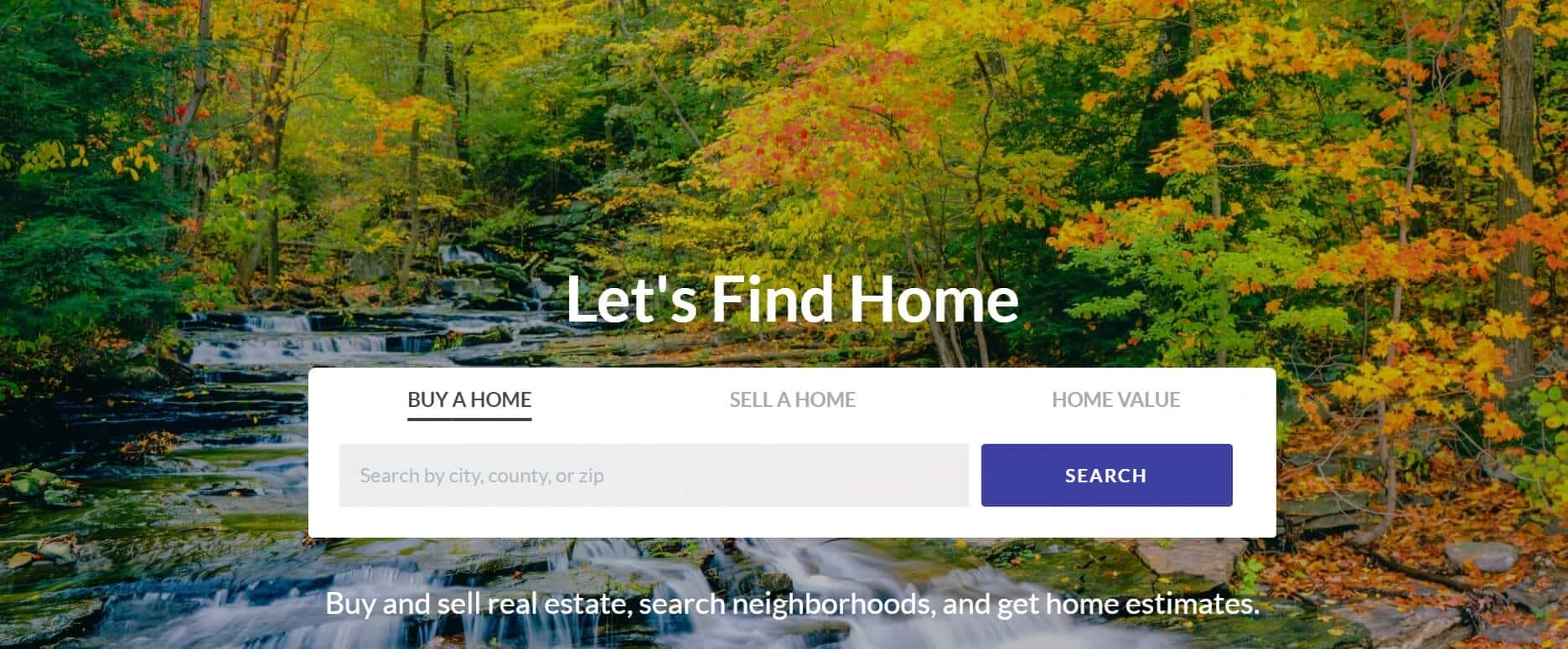The image displays a screenshot from a real estate website, featuring a harmonious blend of functional text elements and a picturesque background. At the center of the screen, a prominent white text reads, "Let's find home," situated above a rectangular interface housing three distinct buttons labeled "Buy a Home," "Sell a Home," and "Home Value." Directly beneath this rectangle, a search text box prompts users with the phrase, "Search by city, county, or zip," accompanied by a vibrant purple button to the right, inscribed with "Search" in white text.

Further down, a descriptive line communicates the website’s offerings: "Buy and sell real estate, search neighborhoods, and get home estimates." The background image enhances the inviting theme of the site, depicting a serene forest scene. Green, yellow, and orange foliage adorns the trees on both sides, while orange leaves gently cover the forest floor. Through the heart of this woodland setting flows a tranquil stream, weaving its way over scattered rocks, adding a sense of natural beauty and calm to the overall visual presentation.